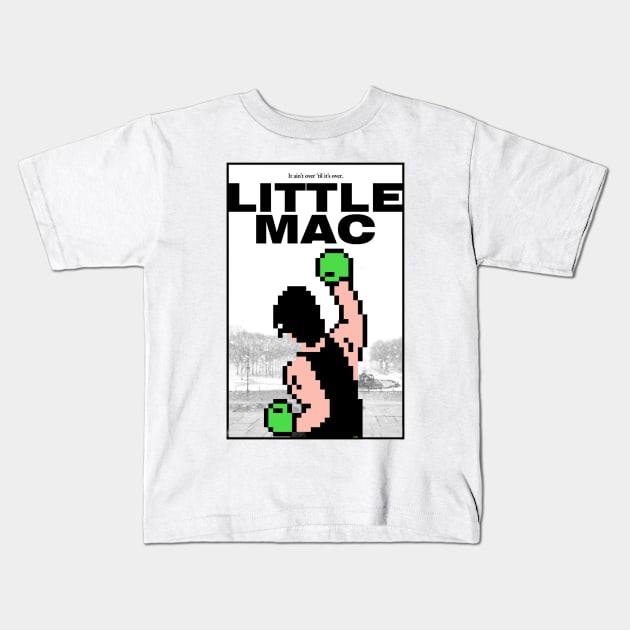The image features a square photograph, approximately four inches by four inches, centered on a plain white short-sleeved crew-neck t-shirt laid against a white background. Dominating the center of the t-shirt’s front is a rectangular print outlined in a thin black border. At the top of this rectangle, the phrase "It Ain't Over Till It's Over" is displayed in a small black Times New Roman font, while directly beneath it, the name "Little Mac" is prominently featured in bold black letters. The main graphic within the rectangle depicts a pixelated boxer, viewed from the waist up, sporting green boxing gloves, a black t-shirt, and black hair. His right arm is positioned close to his side, while his left arm extends forward in a punching motion. The boxer's complexion is light, suggesting he is Caucasian. The background of the graphic includes grayscale illustrations of trees on both the left and right sides, with a white sky above.